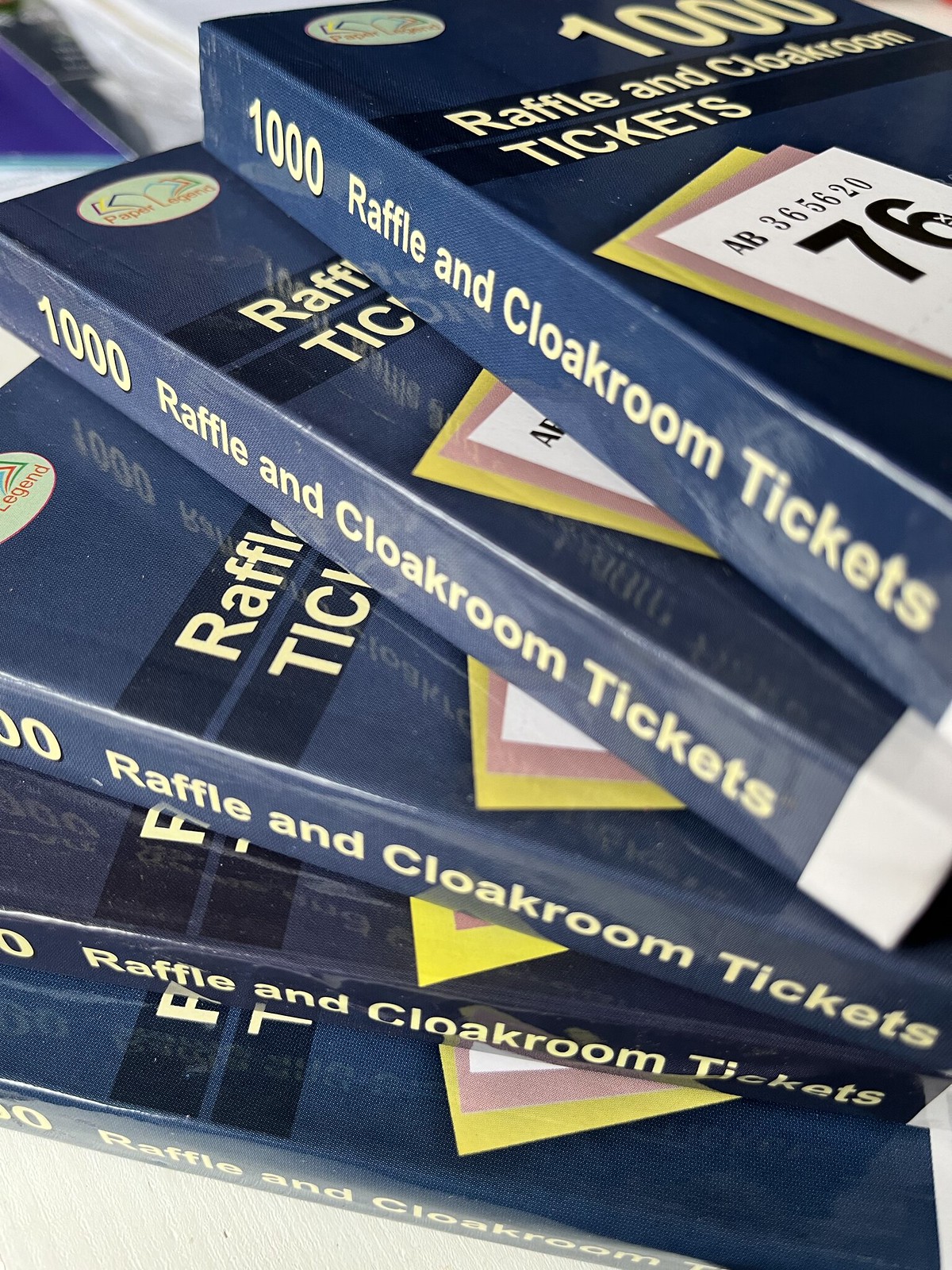In this vertically-oriented photograph, five dark blue books labeled "1,000 Raffle and Cloakroom Tickets" are neatly stacked on a well-lit, tan surface. The books are slightly offset, with each successive book pushed forward a bit more than the one below it. Each book showcases a white emblem on the front, prominently featuring the number '76' along with multi-colored patches of orange, blue, yellow, red, and green. Additionally, there's a sequence of tickets on the top book, with the bottom slip being yellow, the middle slip pink, and the top slip white bearing the black text 'AB365620' followed by a bold '76'. Behind the stack of books lies a pile of documents, adding to the organized yet slightly cluttered composition.